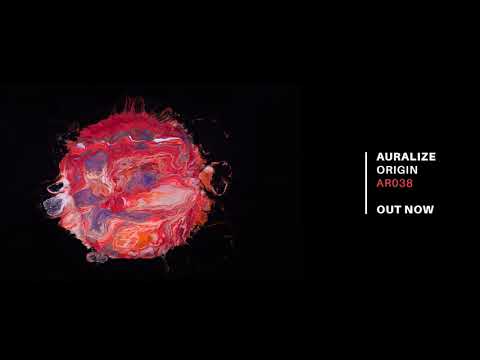The image features a vibrant, irregularly shaped circular splotch on the left side, against a pitch-black background. This vivid shape is filled with swirling layers of red, orange, yellow, pink, purple, and white colors, extending beyond its boundaries and distorting its circular form. There's a small piece protruding on the right center, adding to its uneven, dynamic appearance. On the right side of the image, a vertical white line separates the colorful splotch from white text that reads, in capital letters, "AURALIZE ORIGIN," followed by "AR038" in red, and "OUT NOW" underneath in white. The overall composition suggests a modern, eye-catching digital artwork or a highly magnified microscopic image.